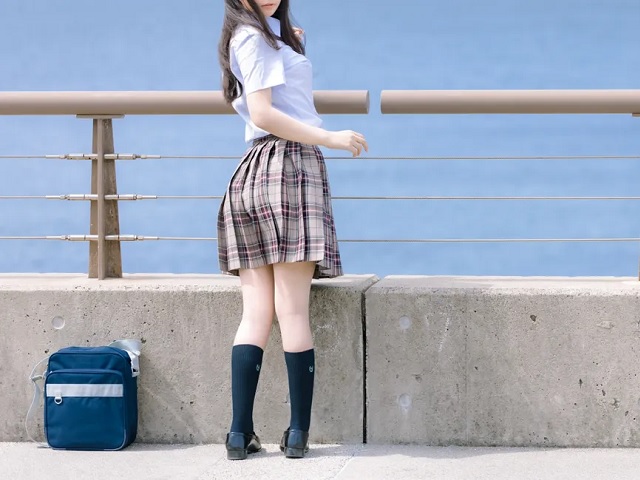The photograph captures a young girl, partially framed so that only her mouth is visible, standing by a cement barrier with a thick, metal railing that features three wire suspensions beneath it. The girl, with long dark hair, is dressed in a short-sleeved white collared shirt neatly tucked into a mid-thigh length brown plaid skirt. She is wearing navy blue knee socks and dark flat shoes. Her stance is coquettish, with her torso turned towards the camera, suggesting a playful invitation. At the bottom left of the image, there is a blue and gray backpack placed on the tan ground near one of the railing supports. The scene is set outdoors under a blue sky, giving a sense of openness and space.